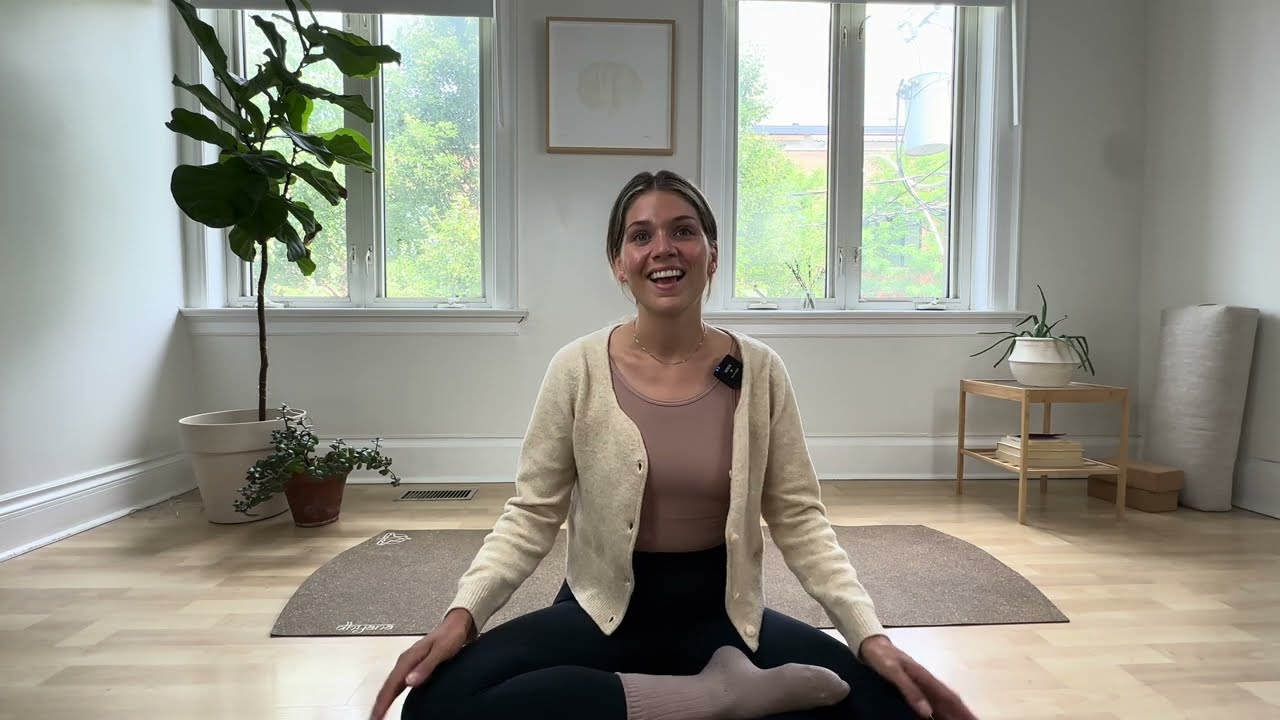A young woman with blondish-gray hair, styled with a middle part, sits cross-legged on a light-colored wooden floor, smiling and appearing to talk to the camera. She wears dark tights, white socks, a beige shirt, and an off-white or beige cardigan. She has a shiny complexion, and a microphone is clipped to the right side of her collar, suggesting she is conducting a tutorial or instructional video. She sits comfortably in front of a yoga mat, placed in the center of a very clean, bright room with white walls and trim. The room features two large sections of windows, through which leaves and tree branches are visible. To the left are two potted plants, while on the right side of the image, there is a small table with another potted plant atop it.